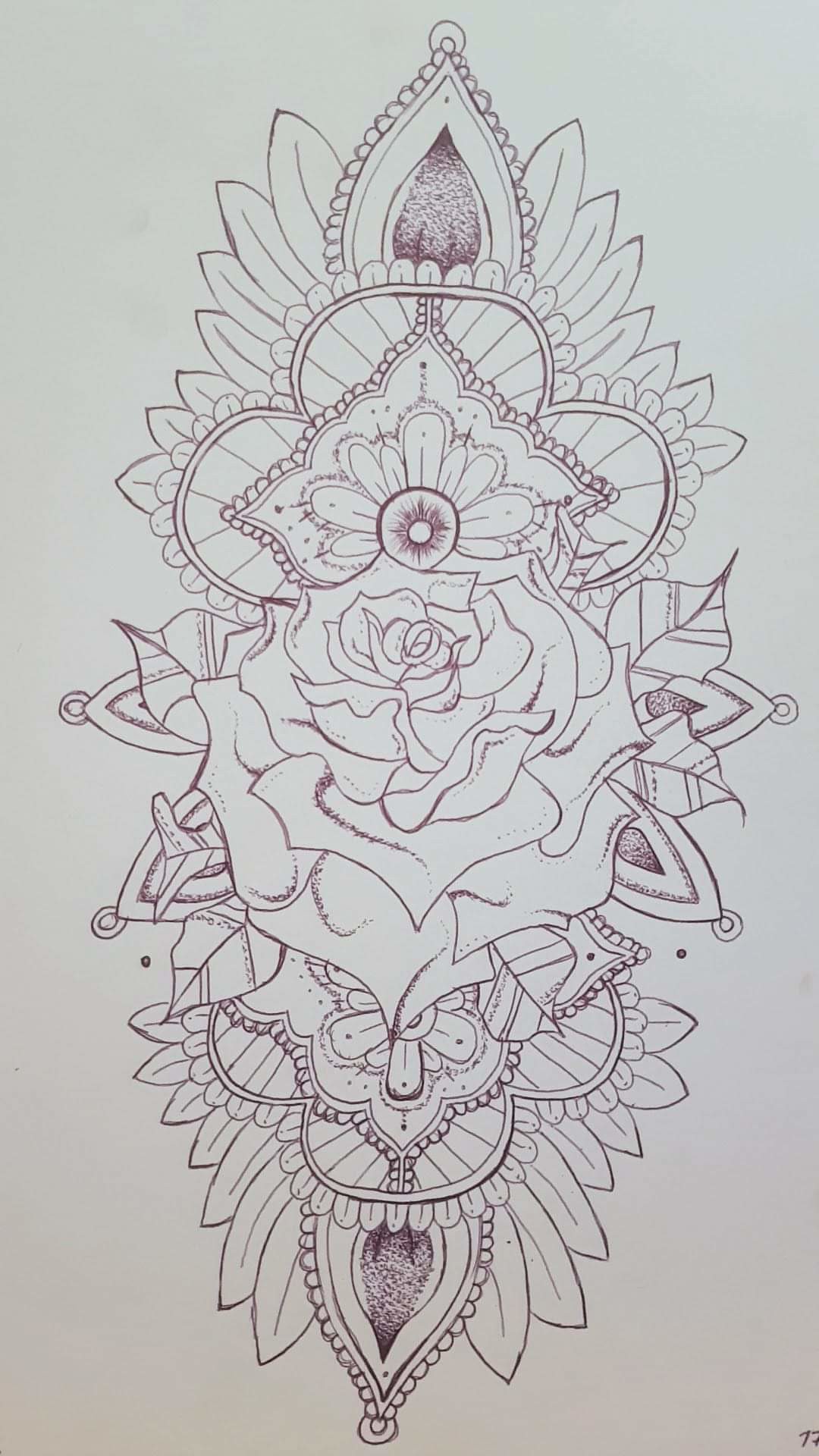This intricately detailed image, possibly a painting or computer-generated drawing, showcases a central rose-like flower with many petals, similar to a carnation, set against a gray or white background with purplish-gray ink. Surrounding the central flower is an elaborate pattern of various leaves and floral designs, including partial drawings of other flowers such as daisies with varying petal counts. This floral motif is framed by ornate, frilly borders at the top and bottom, creating a symmetrical but not perfectly identical mirrored effect. Amongst the sophisticated foliage, subtle differences become apparent upon closer inspection, such as variations in the petal counts and open spaces around the central rose. The entire composition is unified by its floral theme and intricate, repeating patterns.